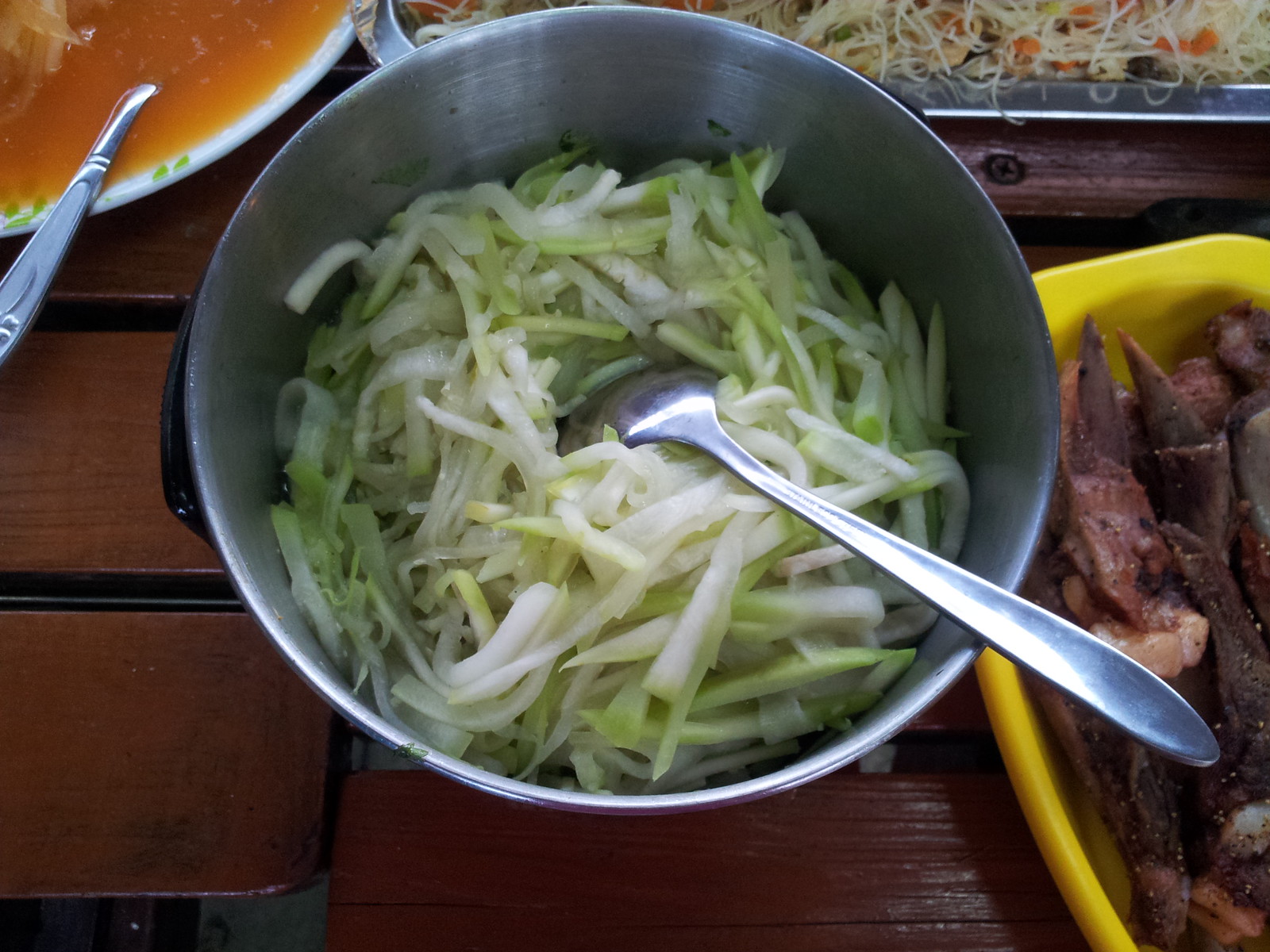The image features a vibrant assortment of foods displayed on a glossy, newly finished wooden table with a visible painted screw. At the center, a metal pot contains chopped onions, leafy green vegetables, and possibly cabbage, with a metal spoon sticking out from the right side. To the left of the pot, a bowl of soup can be seen. Nearby, a partially visible metal tray holds what appears to be thinly grated cheese or possibly angel hair pasta. To the right of the vegetables in the pot, a yellow dish holds cooked pieces of meat, ready to be combined with the vegetables. The overall scene suggests the preparation of an Asian-inspired dish.